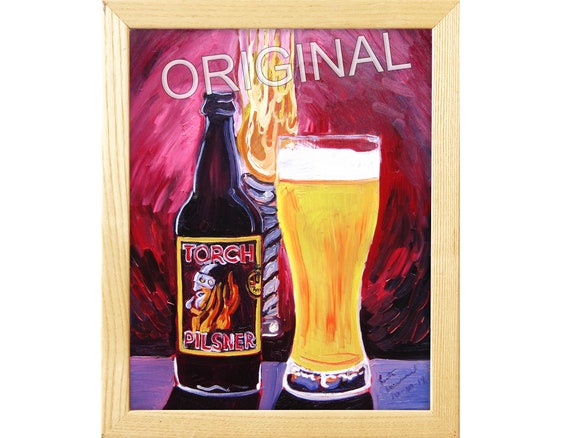This is a framed horizontal painting in a light, natural wood frame. The scene features an uncapped brown beer bottle labeled "Torch Pilsner," prominently displaying a Viking in profile, characterized by a black helmet and an orange beard. Next to the bottle is a clear Pilsner glass, filled with beer and topped with a foam head. The beer and glass rest on a purple table. In the background, there is a torch depicted within red circular brushstrokes, with flames shooting out of the top. "ORIGINAL" is written in large white capital letters diagonally across the top of the image. The background also has a pinkish hue, enhancing the contrast. The painting is signed in the lower right corner, adding a unique touch to the artwork.